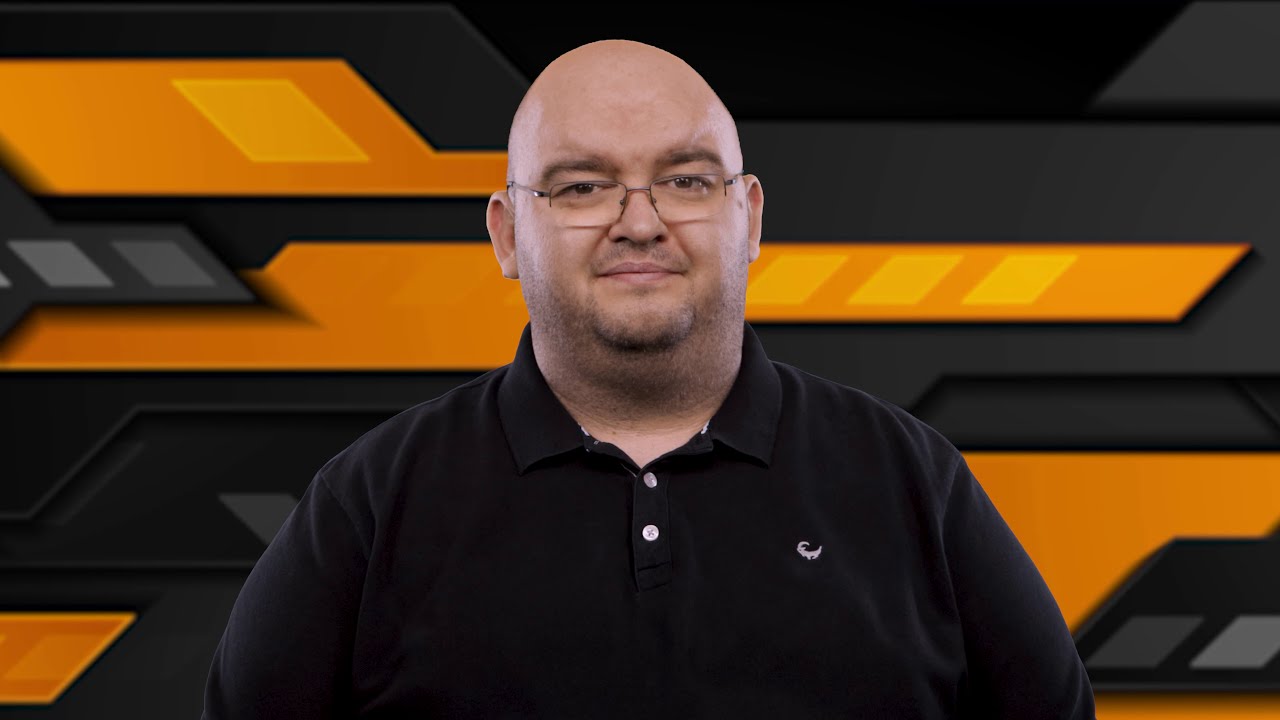This photograph features a stocky, clean-shaven, bald man, smiling as he looks directly at the camera. He is centered in the image, visible from the chest up, wearing thin-framed glasses and a black polo shirt adorned with two white buttons and a small gray logo. The background appears digitally added, showcasing a futuristic, graphically designed orange and black pattern with strong horizontal lines. The scene suggests a high-tech, possibly indoor setting, reminiscent of a modern gaming or presentation backdrop. The overall composition lacks any additional text or objects, highlighting the man as the focal point against the dynamic background.